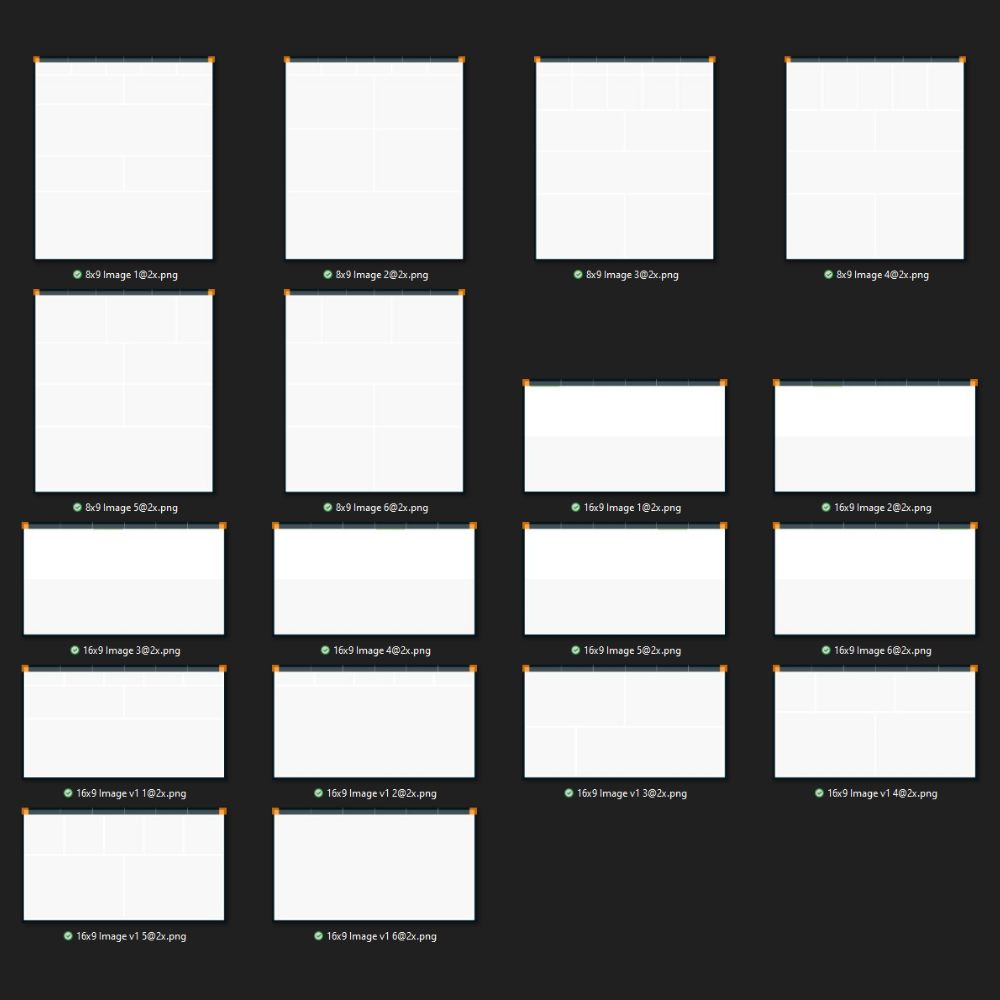The image depicts a grid-like layout with various placeholders for images, each enclosed within a predominantly transparent square PNG container. The background is a solid square, while the placeholders are delineated by white spaces with orange corners on the upper left and right sides. These placeholders are further accentuated by dashed gray lines running across their centers.

In the top row, there are four placeholders, labeled "8x9 image 1 at 2x.png", "8x9 image 2 at 2x.png", "8x9 image 3 at 2x.png", and another similarly labeled placeholder. Each of these has a green circular checkmark icon, characterized by a green circumference, white interior, and a vivid green checkmark, indicating they are complete or verified.

The second row mirrors the top row with four placeholders of similar size, but the two on the right are half the height of the others, aligned at the bottom. This row is labeled in a numerical sequence from "image 5" to "image 8".

Below this, there are two rows of four smaller placeholders each, maintaining consistent spacing. These rows feature a mix of ratios labeled differently, reflecting further segmentation, such as "1x2x" and "16x9".

Lastly, the bottom left corner contains two additional placeholders, continuing the numerical and ratio sequence. The entire layout appears systematically organized into rows and columns, each element meticulously labeled, possibly representing a design template or a storyboard grid.